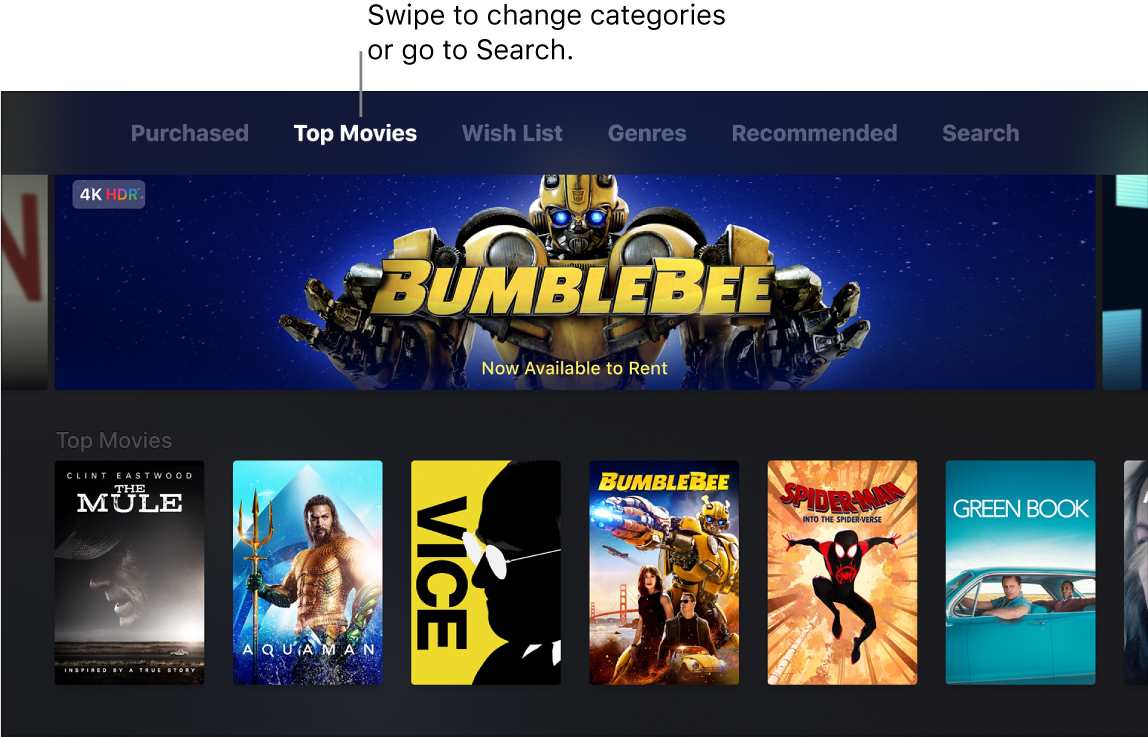At the top of the image, outside the page, there is a white text box with black text stating, "Swipe to change categories or go to search." This directive points to the categories section, which is a series of tabs located at the top of the main page. These tabs, labeled as 'Purchased,' 'Top Movies,' 'Wishlist,' 'Genres,' 'Recommended,' and 'Search' are written in grey on a dark blue background. The 'Top Movies' tab is currently selected, making its text appear white.

Beneath this section, the featured movie advertisement occupies the top left display area. A bold label reading "4K HDR" is prominently displayed, with 'HDR' rendered in a gradient of red, orange, and green. Centrally, the title "Bumblebee" is shown in yellow with a black outline, accompanied by the phrase "now available to rent" in the same yellow font. The background image displays the titular character, Bumblebee, a yellow and black transformer robot with blue eyes, set against a sky that transitions from blue with white stars at the top to black at the bottom.

The bottom portion of the image showcases a selection of six movie thumbnails. From left to right, the films displayed are:
1. "The Mule" by Clint Eastwood, with the subtitle "Inspired by a true story" in white text.
2. "Aquaman," written in white text.
3. "Vice," with the title in black text on a yellow background.
4. "Bumblebee," consistent with the earlier featured advertisement.
5. "Spider-Man: Into the Spider-Verse," with the title in red text.
6. "Green Book," positioned at the far right.